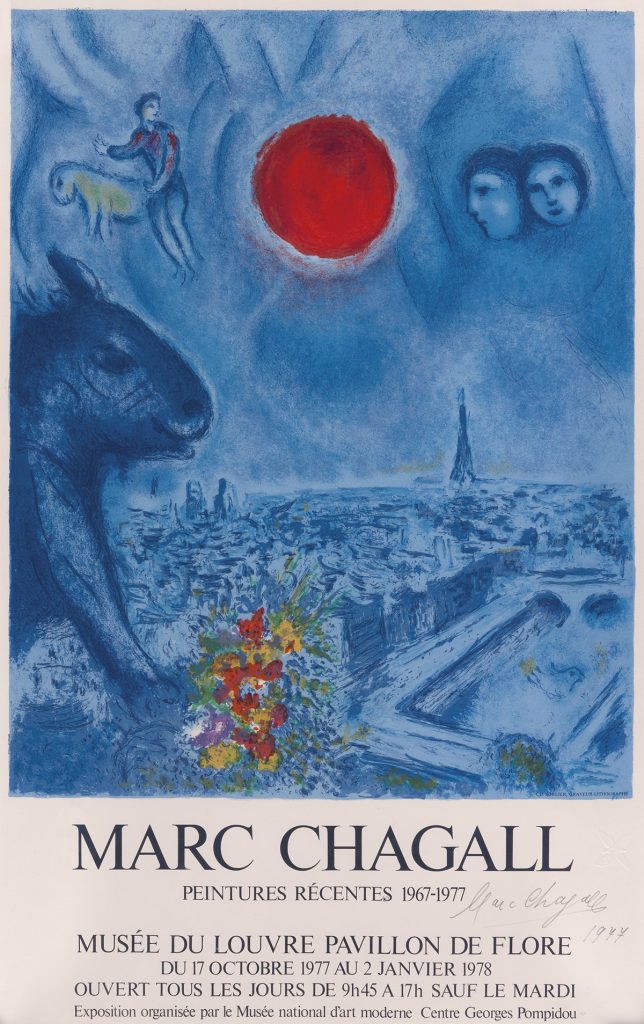This vintage French poster advertises an exhibition of Marc Chagall's works from 1967 to 1977, held at the Musée du Louvre's Pavillon des Fleurs. Rich in detail, the illustration is predominantly blue and features a surreal scene: a red sun or moon is positioned in the top center, flanked by two faces—one gazing at the celestial body and the other facing the viewer. A whimsical cityscape, possibly Paris given the faint outline of the Eiffel Tower, spreads out below, adorned with colorful flowers. To the left, a dark, capybara-like animal emerges, seemingly cradling a bouquet of flowers. Additionally, a person floats in the sky near the sun, accompanied by another indeterminate four-legged mammal, enhancing the dream-like quality of the artwork. The texture is soft and wispy, with fine blue brush strokes bringing the fantastical scene to life.